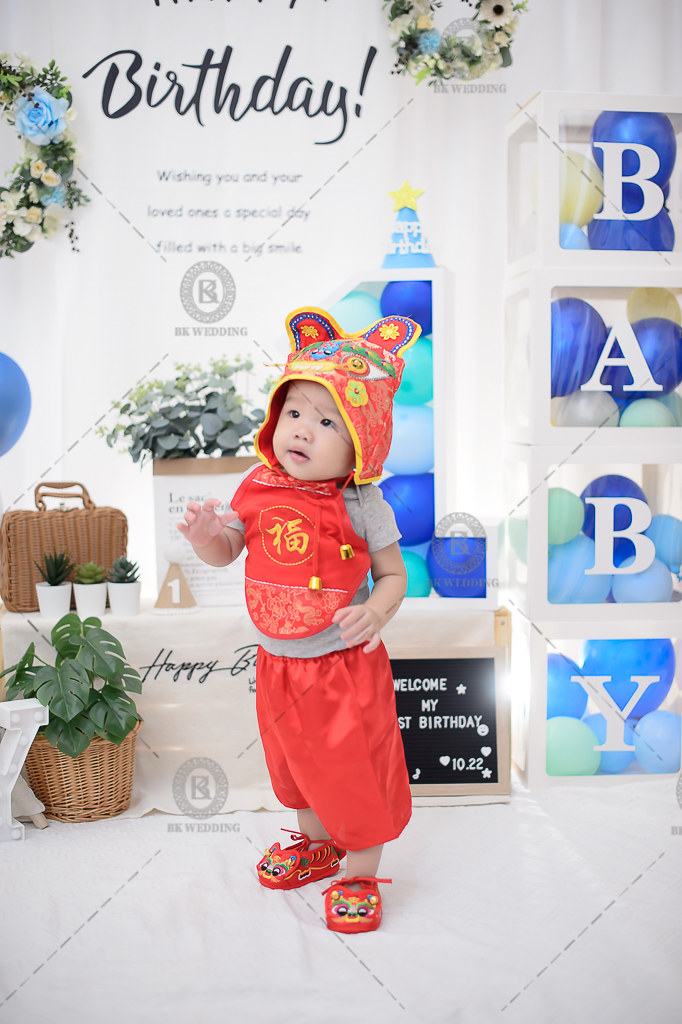The image showcases a young Asian child, likely celebrating their first birthday, standing on a white floor. The child is dressed in a predominantly red outfit, featuring shiny red poofy pants, red moccasin-like shoes with a colorful cat face design, and a deep red bib adorned with a golden Chinese symbol over a gray t-shirt. Topping off the outfit is a red hat with gold-adorned ears resembling a dragon. The child looks up to the left with curiosity.

Prominently in the background, the top of the wall displays "Birthday" in black letters, and below it, a heartfelt message reads, "Wishing you and your loved ones a special day filled with a big smile." To the right of the child, four transparent white blocks stacked vertically spell out "B-A-B-Y" in white letters against a dark blue backdrop, with blue balloons nestled inside each block. Further behind the child, a black sign with white lettering reads, "Welcome my first birthday," and is dated "10.22." Intricate details like shelves adorned with more balloons and a wicker basket with a green leafy plant add depth to the celebratory setting.